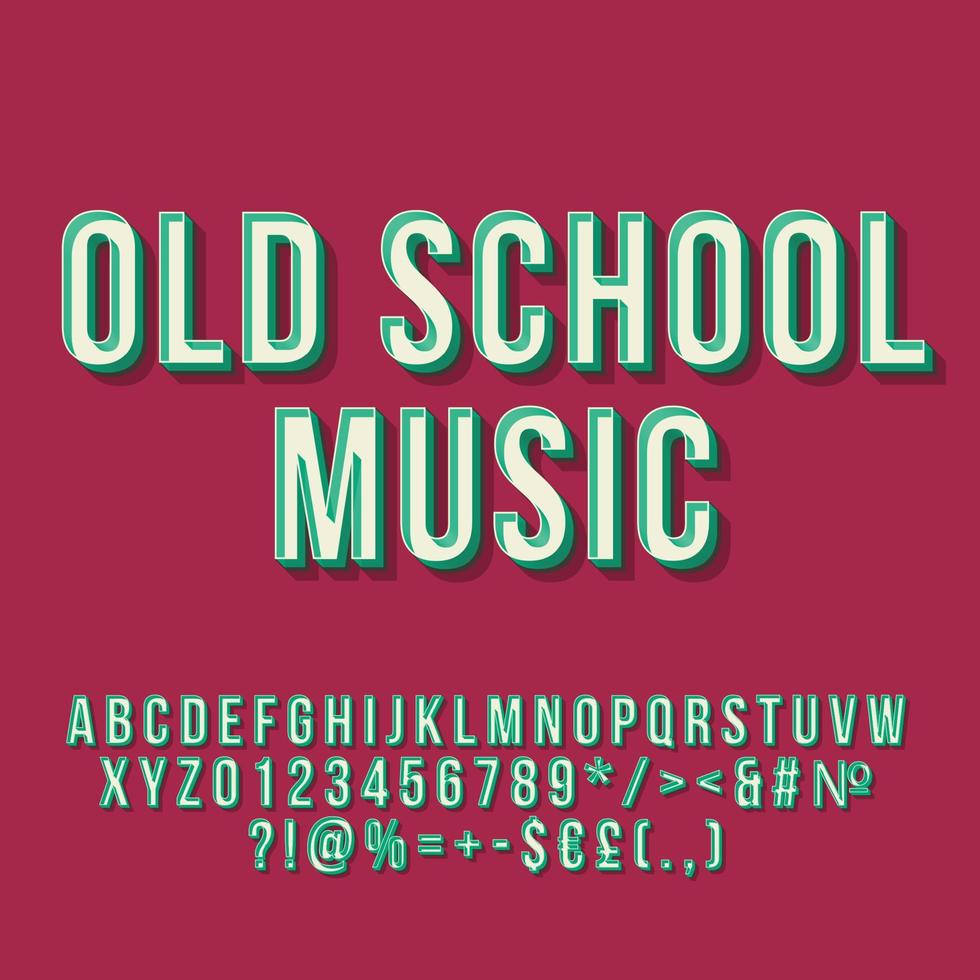The image features a square format with a background in dark burgundy red, tinged slightly with pink. Dominating the top two-thirds of the image are the words "OLD SCHOOL MUSIC" written in bold, white, all-caps letters, accented with green edges and shadowing that gives them a floating, three-dimensional appearance. Below this prominent text, occupying the bottom third, is a detailed character set designed in the same blocky, three-dimensional style. This segment includes the full alphabet from A to Z on the first line, followed by the numbers 0 through 9 and a variety of special characters such as asterisk, forward slash, greater than and less than signs, ampersand, hashtag, N-O abbreviation, question mark, exclamation point, at sign, percent sign, equal sign, plus sign, minus sign, dollar sign, another currency symbol, pound sign, parentheses, period, and comma. This comprehensive character demonstration is spread across two nearly full rows and a shorter centered segment at the bottom, maintaining the cohesive 3D look throughout.